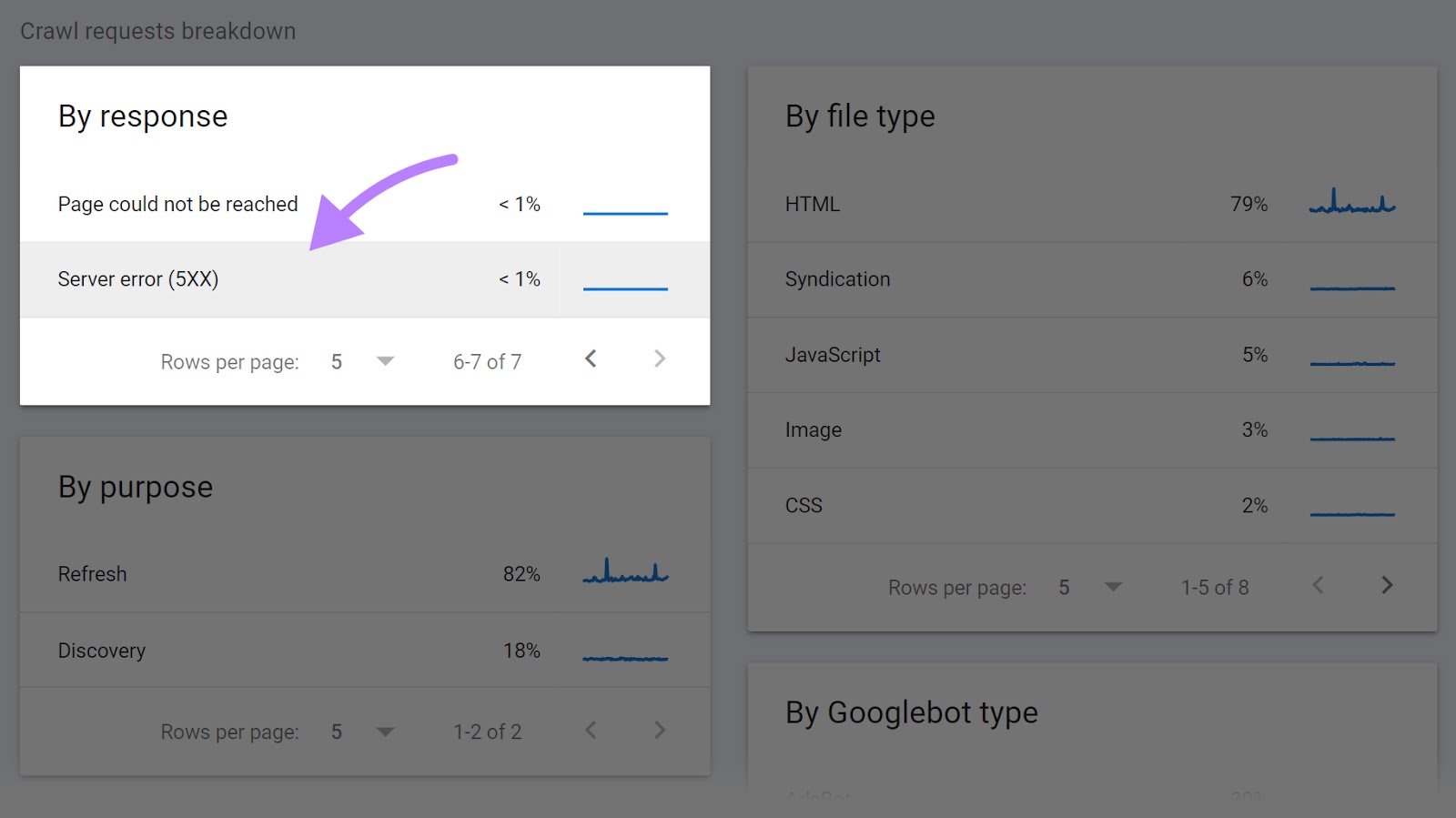In the image, there is a screenshot displaying three distinct sections, with one box highlighted and more prominent than the others. The highlighted box, located at the top left, is labeled “By Response”. Within this box, the text “Page Cannot Be Reached” is shown next to a purple arrow pointing to the right. Beneath this, it states “Server Error 5 of 5xx” with an adjacent indicator showing “> 1%”. To the right of this highlighted box, a horizontal blue line runs across the screen.

The second column in the image is light gray and features pagination details at the bottom, specified as “Rows per page 5” and “6 out of 7 of 7”. Below this, there is another section titled “By Purpose,” offering two options: “Refresh” and “Discovery.” Refresh has an 82% rate, while Discovery stands at 18%. Each percentage is accompanied by a graph resembling a heart rate monitor line.

To the right of the “By Purpose” section, there's a category named “By File Type” that lists five file types along with their respective percentages: HTML (79%), Syndication (6%), JavaScript (5%), Image (3%), and CSS (2%).

At the very bottom of the image, the text “By Googlebot Type” is displayed in black. The entire image has a gray background, except for the prominent box in the top left corner that stands out more noticeably than the rest.